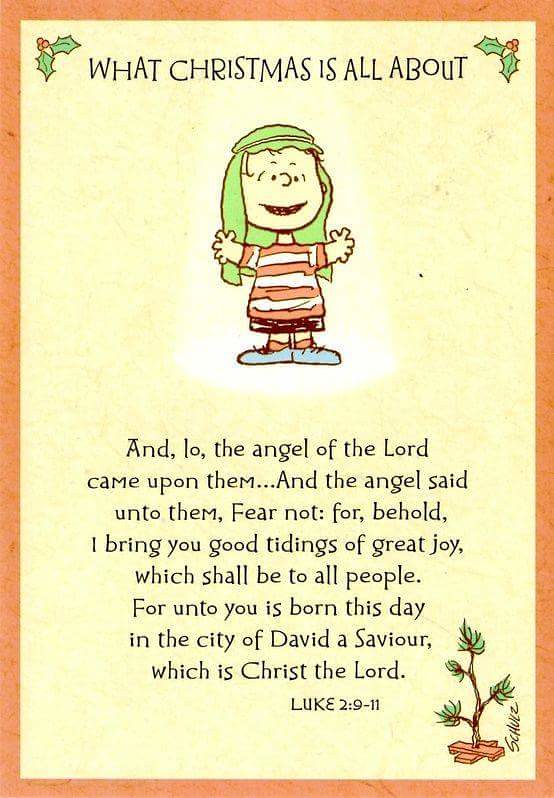This detailed holiday card features a nostalgic Christmas design centered around the beloved character, Charlie Brown, from the Charlie Brown Christmas television special by Charles Schulz. The card has a light yellow-green background, bordered by a thin, dark orange line. At each of the top corners, there is a holly graphic with two green leaves and red berries. Centered at the top, between these holly decorations, the text "WHAT CHRISTMAS IS ALL ABOUT" is prominently displayed in bold, black capital letters.

Beneath this headline, Charlie Brown stands in the top half of the card, facing the viewer with his arms open wide. He is donning a green hat and his classic black and white shirt paired with blue shoes. Below Charlie Brown, a biblical passage from Luke 2:9-11 is written in black text, which reads: "And lo, the angel of the Lord came upon them, and the angel said unto them, Fear not, for behold, I bring you good tidings of great joy, which shall be to all people. For unto you is born this day in the city of David a Savior, which is Christ the Lord."

At the bottom right corner, a tiny depiction of the iconic Charlie Brown Christmas tree with green needles and a lone red ornament stands next to the signature of Charles Schulz.